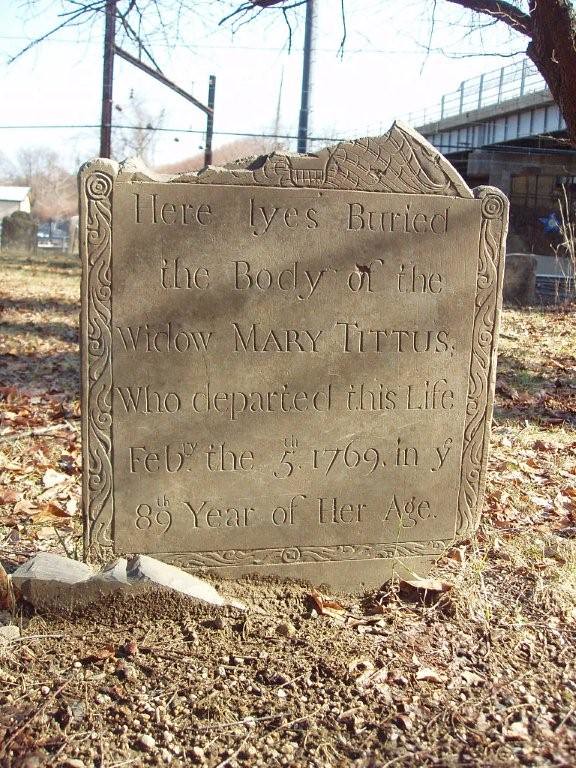In the foreground of the image lies an aged, square-shaped gravestone, partially broken at the top. The gravestone is brown and contains the text: "Here lies buried the body of the widow Mary Titus who departed this life Feb 5, 1769 in Y 89th year of her age." The stone also features curved designs along its borders. Resting on ground covered in brown soil and dried leaves, the grave marker is clearly legible despite its weathered appearance and discoloration. The scene is set in a poorly maintained area with scattered foliage, indicative of the fall or early winter season. In the background, bare tree branches and a blue sky are visible, alongside modern elements such as rooftops, telephone poles, and a freeway overpass, highlighting the tombstone's presence in an otherwise developed neighborhood. This centuries-old gravestone, marking the final resting place of Mary Titus, stands as a historical relic amid its evolving surroundings.